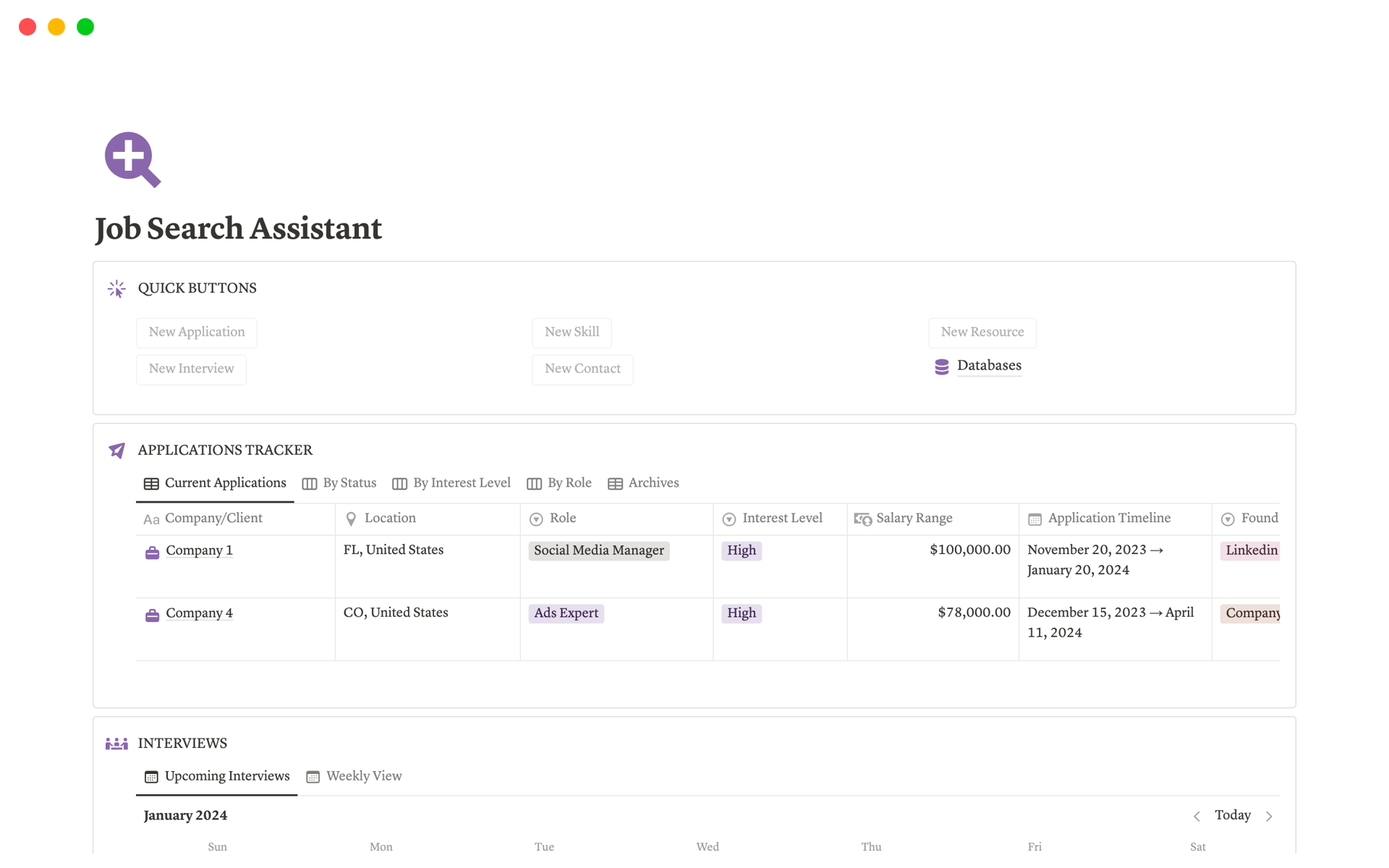**Caption:**

A detailed screenshot of a job search application on a MacBook screen. The familiar red, yellow, and green dots in the top left corner indicate an active window. Although the URL is not visible, the interface reveals a webpage for a job employment platform named "Job Search Assistant." At the very top, there's a distinctive purple magnifying glass icon with a white plus symbol at its center.

Below the header, several informative cards are displayed. The first card, titled "Quick Buttons," offers clickable options for various actions: New Application, New Interview, New Skill, New Contact, New Resource, and Databases. Beneath this, the "Applications Tracker" card features five tabs: Current Applications, By Status, By Interest Level, By Role, and Archives, with "Current Applications" currently selected. This section lists two different job entries, providing details about the companies applied to.

Further down, the "Interviews" section is revealed with two tabs: Upcoming Interviews and Weekly View. The "Upcoming Interviews" tab is selected, showcasing a calendar for January 2024, with days spanning from Monday to Saturday. Today's date is highlighted, giving a clear view of the user's upcoming schedule.